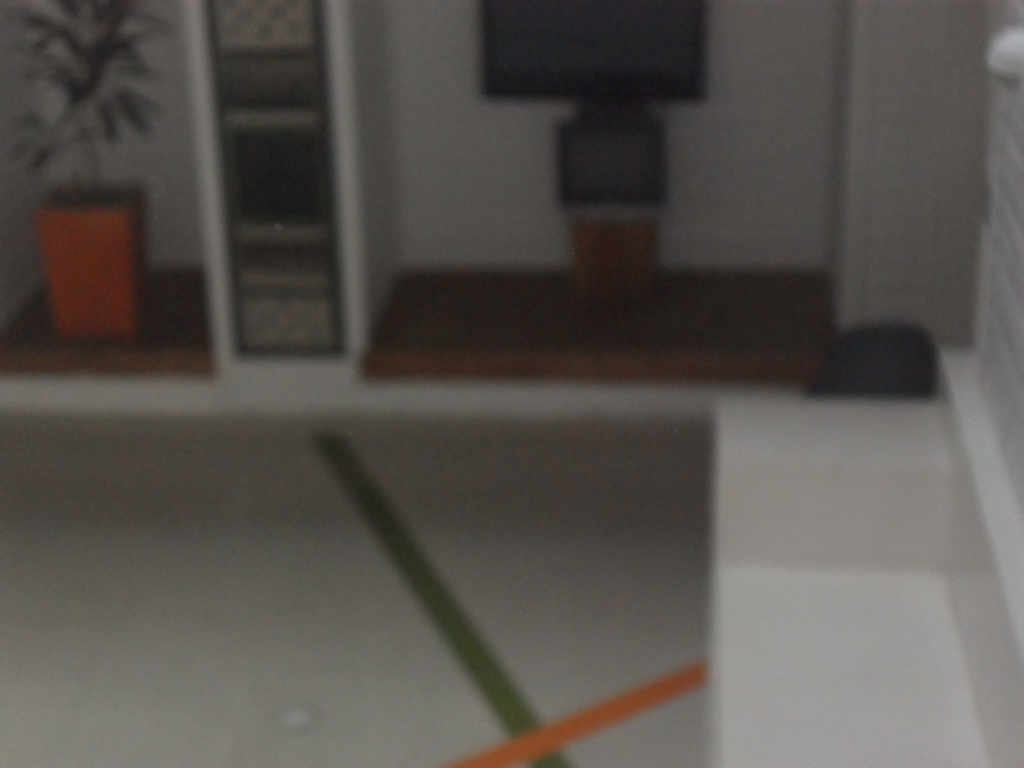This image depicts a white room, captured in a blurry and dark setting, creating a somewhat obscured view. The room features countertops positioned at the front and right sides. The flooring is white and is accentuated by a single green stripe running perpendicular to an orange stripe. A potted plant in an orange pot is situated toward the left. On the right, there is a TV screen mounted on a wooden beam, accompanied by a smaller TV screen nearby. The walls are adorned with white tiles, adding to the monochromatic aesthetic of the room.